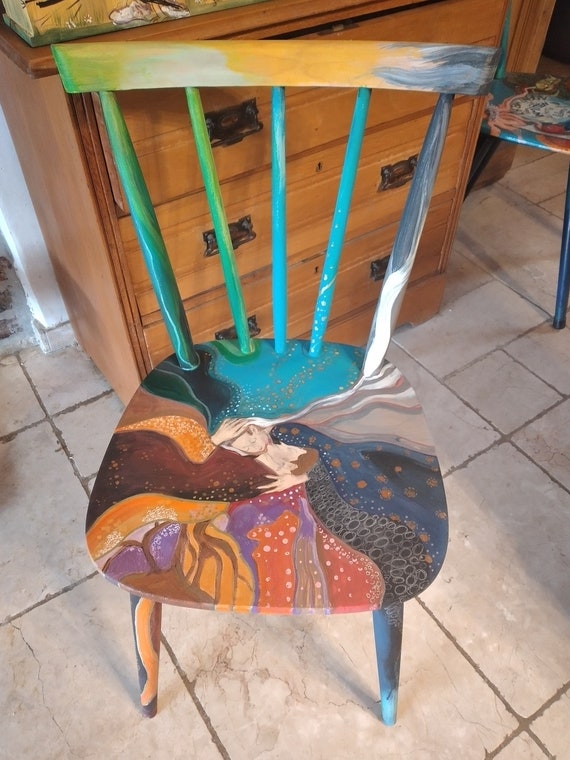The photograph showcases a repurposed wooden dining chair, intricately painted with a vibrant and fantastical design. The focal point of the chair is its flat wooden seat, which features a stylized and romantic painting of a man and a woman embracing each other's heads. This artwork, reminiscent of Klimt’s ornate style, is surrounded by various fantastical trees and a night sky at the upper part. The painting on the seat predominantly uses colors such as blue, brown, red, black, orange, and purple, contributing to its whimsical charm. The backrest, characterized by several radial holes, is also richly painted in different colors, primarily blue and green. Each leg of the chair, as well as the spindles of the backrest, display unique designs and colors, including dots, swirls, and lines, enhancing the chair’s funky and eclectic aesthetic. The scene is set on a floor of large gray tiles, grouted with gray, in what seems to be a home environment. In the background, there is a light brown wooden dresser with three drawers, each equipped with two handles, adding to the domestic ambiance of the image.